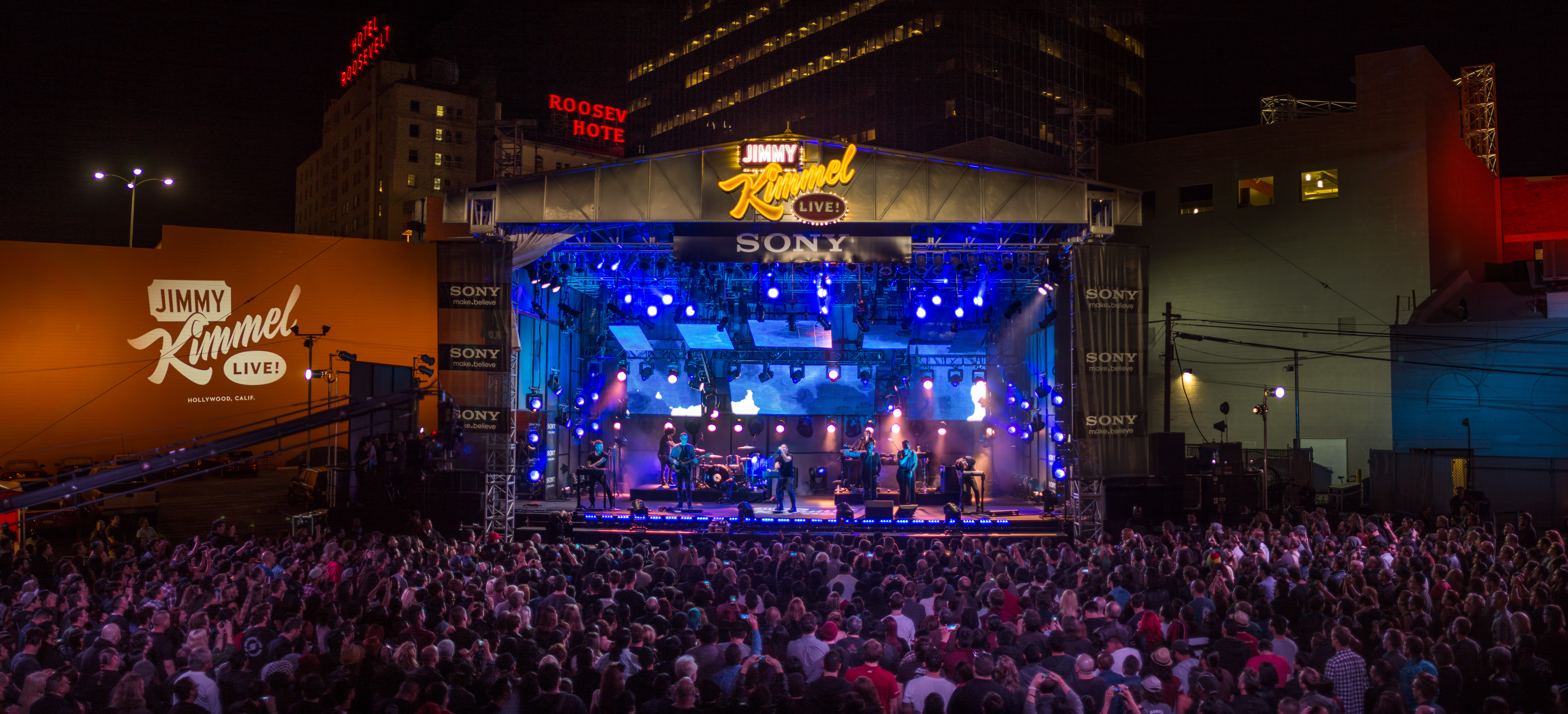The image depicts an outdoor concert scene from Jimmy Kimmel Live, featuring a large stage set against a nighttime cityscape. The stage is bathed in blue and white lights, illuminating seven standing musicians who appear to be performing. Above the stage, a sign reads "Jimmy Kimmel Live," with "Sony" displayed underneath it on a black background. The stage is framed by curtains adorned with the Sony logo.

In the background, several buildings are visible, including the recognizable Roosevelt Hotel. The hotel's red-lettered sign is partially obscured by a white building. To the left, an orange wall bears the "Jimmy Kimmel Live" logo. The crowd in front of the stage is substantial, possibly numbering in the hundreds, filling the space from left to right. Elements like a light post with four lights and various red and blue structures add to the dynamic urban backdrop.